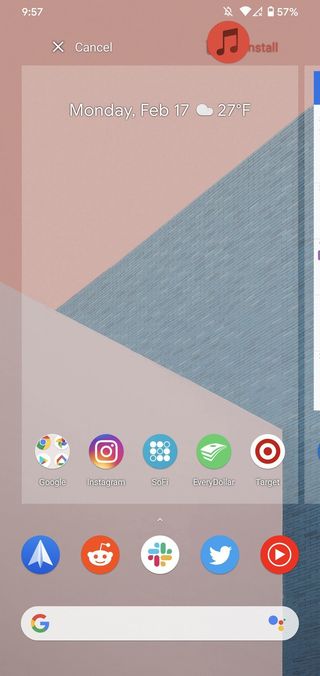The image is a screenshot of a smartphone home screen. The background is divided into multiple sections with varying colors. Starting from the left side and moving halfway down, then angling down to the right about an inch, and then going up to the right about two inches from the top corner, the background is a dark pink color. On the right side, starting about two inches from the left and moving down and back over to the right about two inches, and then further down off the bottom, the background color resembles blue denim. The lower left section is a lighter pink.

At the top of the screen, the time is displayed on the left as 9:57, while the battery percentage is shown on the right at 57%, accompanied by the battery icon. The Wi-Fi icon indicates a full connection, but there are no signal bars for cellular reception. Additionally, the sound icon is muted, as indicated by a line through it. Below the time, there's a horizontal white "X" next to the word "Cancel" in white. 

To the right side, there's a prominent red circle with a black music note inside it. Next to this, the text "INSTALL" appears in red. A semi-transparent pop-up tab allows partial visibility of the background. At the top of this tab, it states the date "Monday, FEB 17," with a small white cloud icon next to the temperature, which is 27°F.

The bottom part of the pop-up tab shows four icons with corresponding labels: Google, Instagram, SoFi, and EveryDollar, followed by a fifth icon, Target. Outside of the pop-up, four more app icons are visible: a blue icon with a white paper airplane, Reddit, Slack, and Twitter. Additionally, there's a red circle with a white border and a play button inside it. At the very bottom of the screen is a gray search bar.